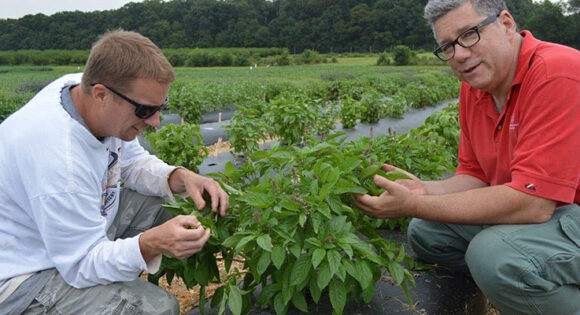This photograph captures two men, an older gentleman and a younger man, immersed in observing a plant with understated flowers, likely in a farming or botanical setting. The background reveals a lush, expansive field bordered by green, leafy trees, suggesting a well-maintained farm environment. The rows of plants, possibly herbs, are neatly aligned and covered with black tarp, with narrow pathways in between that are filled with water.

The older man, positioned on the right and facing the camera, sports a short-sleeved red polo shirt paired with green army cargo pants. On the left, the younger man, wearing sunglasses, a long-sleeved white shirt, and gray pants, has short light brown hair. Their contemplation of the plant reflects their potential roles as botanists or herb farmers, engaged in the careful cultivation and study of their crops. The sky appears overcast, indicating a cloudy day without rain, adding a serene ambiance to their focused interaction.